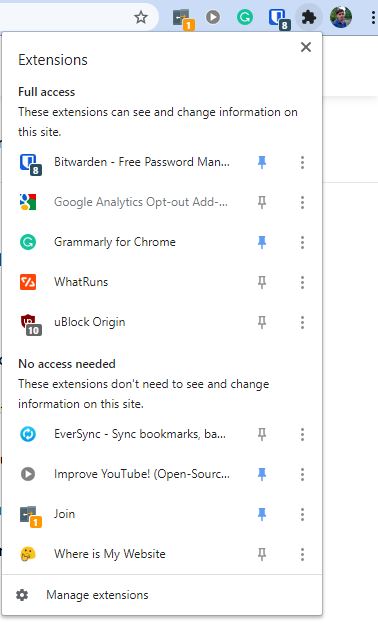A detailed image description:
The image showcases a vertical, rectangular browser extension manager interface. At the very top of the interface, there is a light blue ribbon. Within this ribbon, starting from the left, there is a search box accompanied by a star icon to its right, suggesting a favorite or bookmark feature. Next to this, several functional icons are displayed. Toward the far right of the ribbon, there is a user profile photo depicting a young man with dark hair and darker skin.

Below the ribbon, the main section of the extension manager begins. It is divided into two sections, labeled "Full access" and "No access needed."

At the top of the main section, in dark grey print, appears the title "Extensions." Directly beneath it, in bold print, is the header "Full access," followed by a description: "These extensions can see and change information on this site." Listed under this section are several extensions:
1. **Bitwarden** (Free Password Manager) - Pinned
2. **Google Analytics Opt-out Ad** - Pinned
3. **Grammarly for Chrome** - Pinned
4. **WhatRuns**
5. **uBlock Origin**

Following this list, the header changes to "No access needed," with a subheading explaining that "These extensions don't need to see and change information on this site." The extensions listed here include:
1. **EverSync**
2. **Improve YouTube** - Pinned
3. **Join** - Pinned
4. **Where is my website**

At the very bottom of the extension manager, there is an option to "Manage extensions," accompanied by a settings icon to the left of this text.